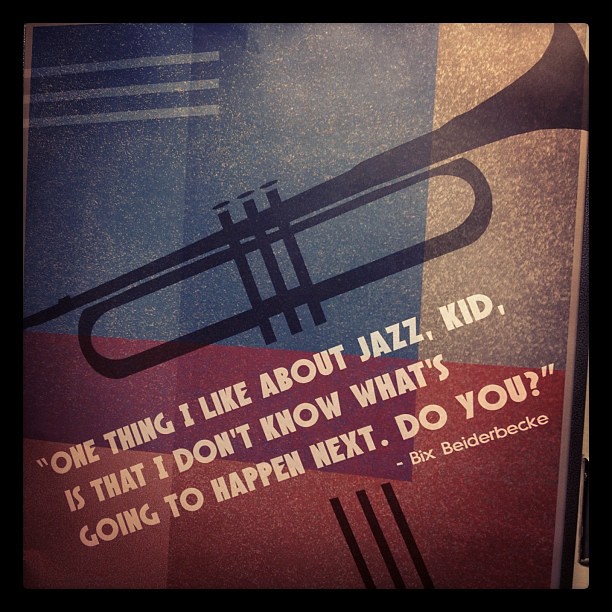The image is a detailed photograph of a vibrant poster featuring a prominent black silhouette of a trumpet. The trumpet is artistically illustrated and positioned diagonally at about a 45-degree angle, stretching across the poster yet not entirely fitting within the frame. The background is geometric, made up of overlapping colored rectangles in shades of blue, red, yellow, and green, creating a visually engaging, grainy texture where the colors mix. Overlaying this dynamic composition is a bold, white sans serif font that says, "One thing I like about Jazz Kid is that I don't know what's going to happen next. Do you?" This quote is attributed to someone named Bix Beiderbecke, with the name written below the quote in the same white sans serif font, but only the first letters of each word capitalized.